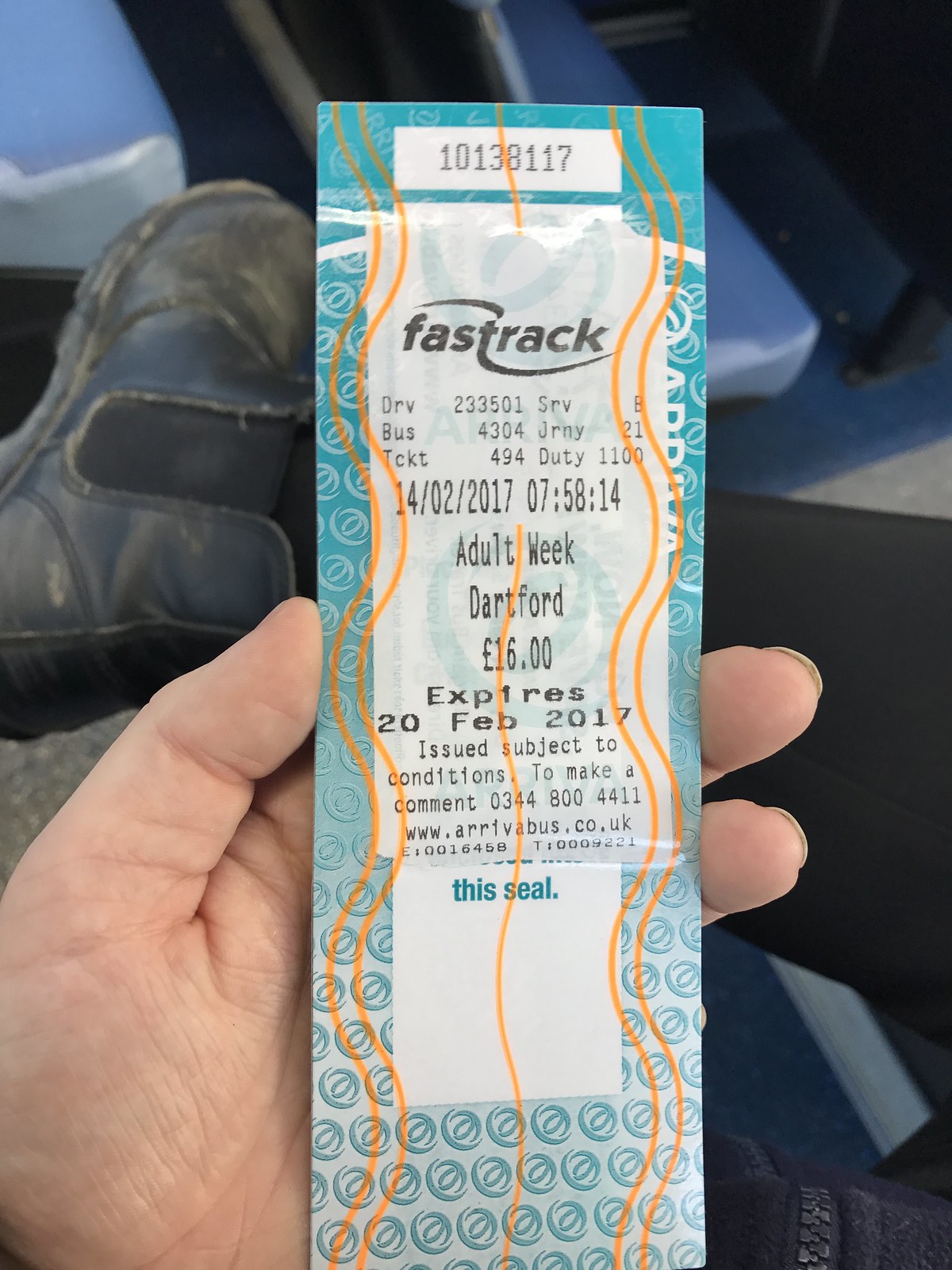A detailed photograph captures a person's hand holding a tall, thin bus ticket issued by Fast Track. The ticket, bordered in blue with circular symbols and orange vertical squiggly lines, features an eight-digit serial number, 10138117, at the top. Below, in black text, are various details including the service name "Fast Track," abbreviated terms (DRV, bus, ticket, serve, JRNY, duty) each followed by a number, and specifics such as "adult week, Dartford, 16 pounds." The ticket is dated 14-02-2017 at 7:58 AM and expires on 20 February 2017. The issuer's conditions, a phone number, and a URL are also noted.

In the image, the holder's right leg is crossed over the left knee, revealing part of their jeans, a jacket zipper, and a black boot. The scene is illuminated by daylight, likely taken during a bus ride as the floor of the bus and edges of seats are visible, suggesting traveling at an early morning hour. The person, possibly a woman considering the longer fingernails and minimalist, possibly feminine boot, presents a serene moment in transit.